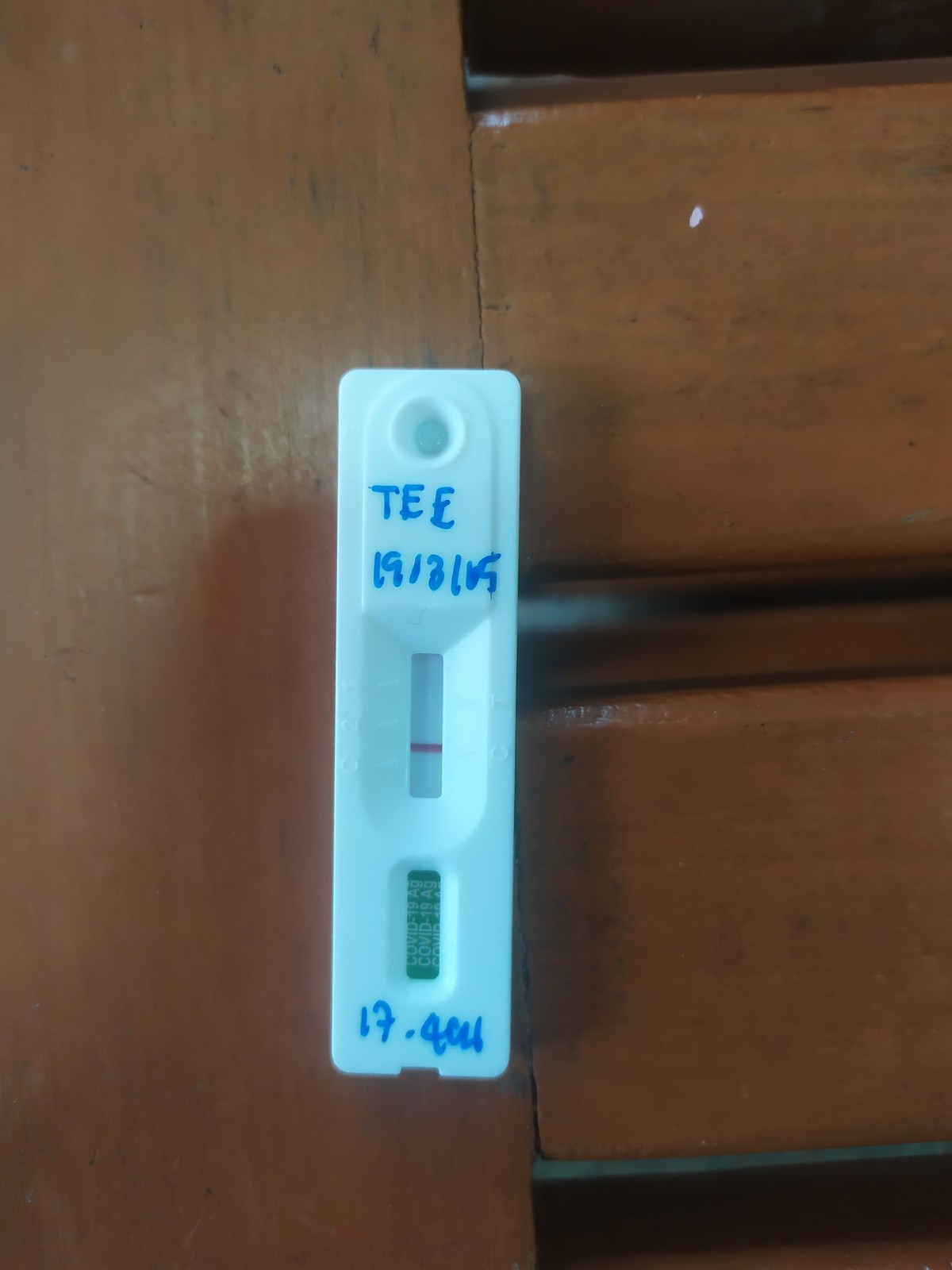This image showcases a white pregnancy test stick positioned on a brown piece of furniture, possibly a dresser or desk. The pregnancy test, identified with the code "TE1913809," features a rectangular window in the center displaying a faint pink horizontal line. Below this window, the number "17" is clearly visible, though the text following it is indistinguishable. All the inscriptions on the stick are written in a blue marker.